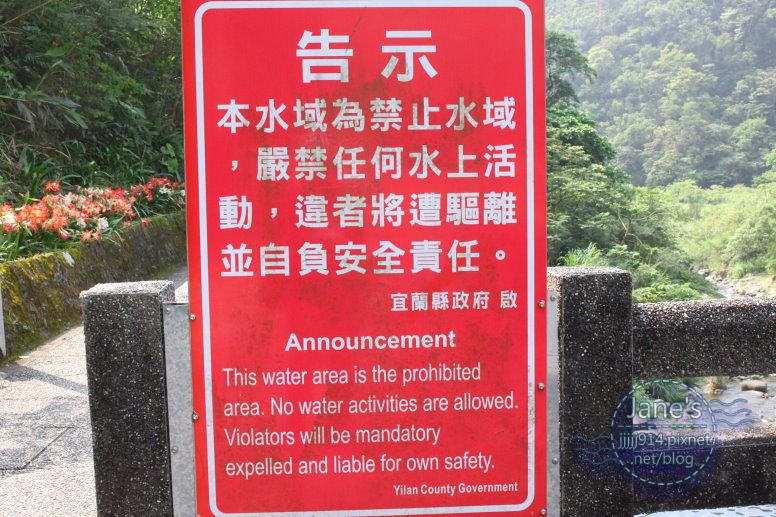The photograph captures a tranquil outdoor scene dominated by a red rectangular sign in the foreground. The sign bears Asian characters at the top and translates to English below, stating: "Announcement. This water area is the prohibited area. No water activities are allowed. Violators will be mandatory, expelled, and liable for own safety." At the bottom, it is marked by the Yan (or Yilan) County Government. The sign stands in front of a stone fence, beyond which lush green trees and a river can be seen. On the right side, a partial view of a walkway features flowers and additional trees lining it. The detailed setting includes a mix of green foliage and vivid orange flowers, indicating a maintained, aesthetically pleasing outdoor environment. A caption in the small right corner of the image reads, "Jane's JJJ918picsnet.net/blog," adding a personal or professional touch to the documenter of the scene.